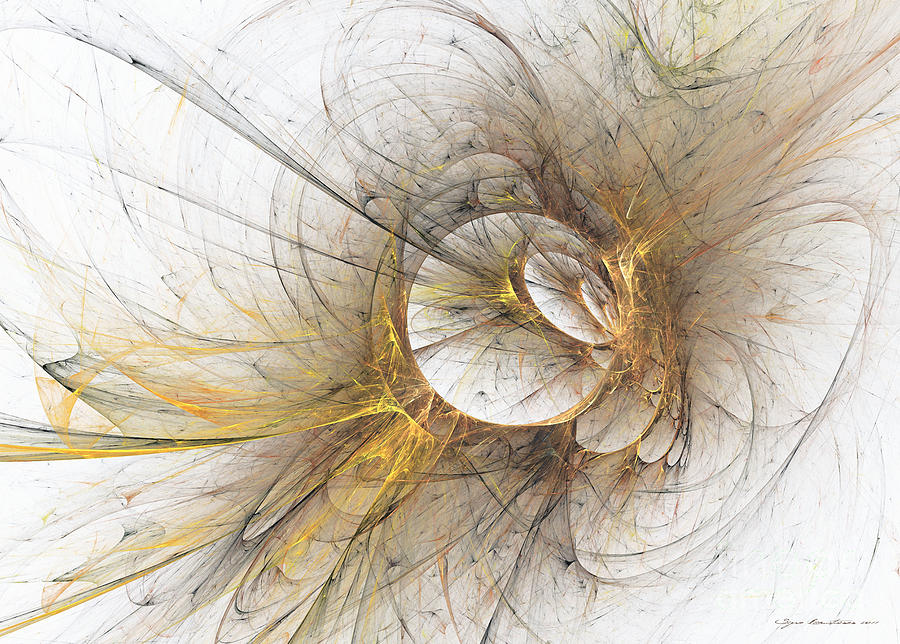This image depicts an abstract, mixed-media artwork with a predominantly white background, resembling a wide horizontal canvas. Central to the piece are intricate circular formations that evoke the appearance of a "big cobweb" made up of varying shapes, some of which are reminiscent of flower petals. This central motif is densely packed with vibrant colors, especially black, yellow, orange, and white, with touches of red and brown. The streaks originating from the center vary between straight lines and looping curves, adding dynamic movement to the composition. The top left and bottom right corners are largely white, with bursts of colors creating splotches and streaks, mainly in black and yellow, with hints of green and red especially in the bottom left area. A cursive black signature is located in the bottom right corner, but remains illegible.